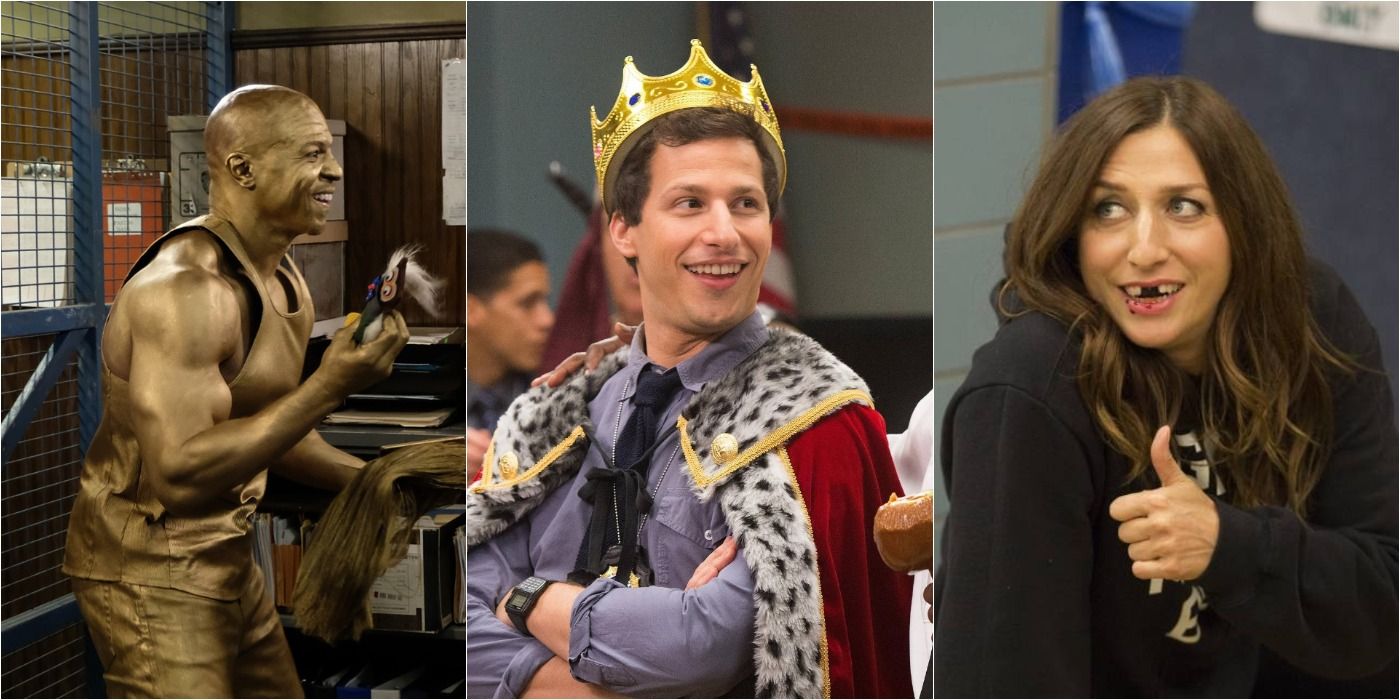This is a triptych featuring comedic scenes from the TV show Brooklyn Nine-Nine. On the left, Terry Crews, painted entirely bronze and dressed in a tank top, is smiling in profile, resembling a trophy. In the center, Andy Samberg, known on the show as Jake, combines his police uniform with a regal costume, wearing a plastic gold crown and a red, fur-trimmed cape. He stands smiling amidst a backdrop of other people. On the right, Chelsea Peretti's character, with long brunette hair and a black sweatshirt, gives a thumbs up while humorously displaying what seems to be missing front teeth. Each character’s unique costume and expression contribute to the overall humorous and whimsical nature of the images.